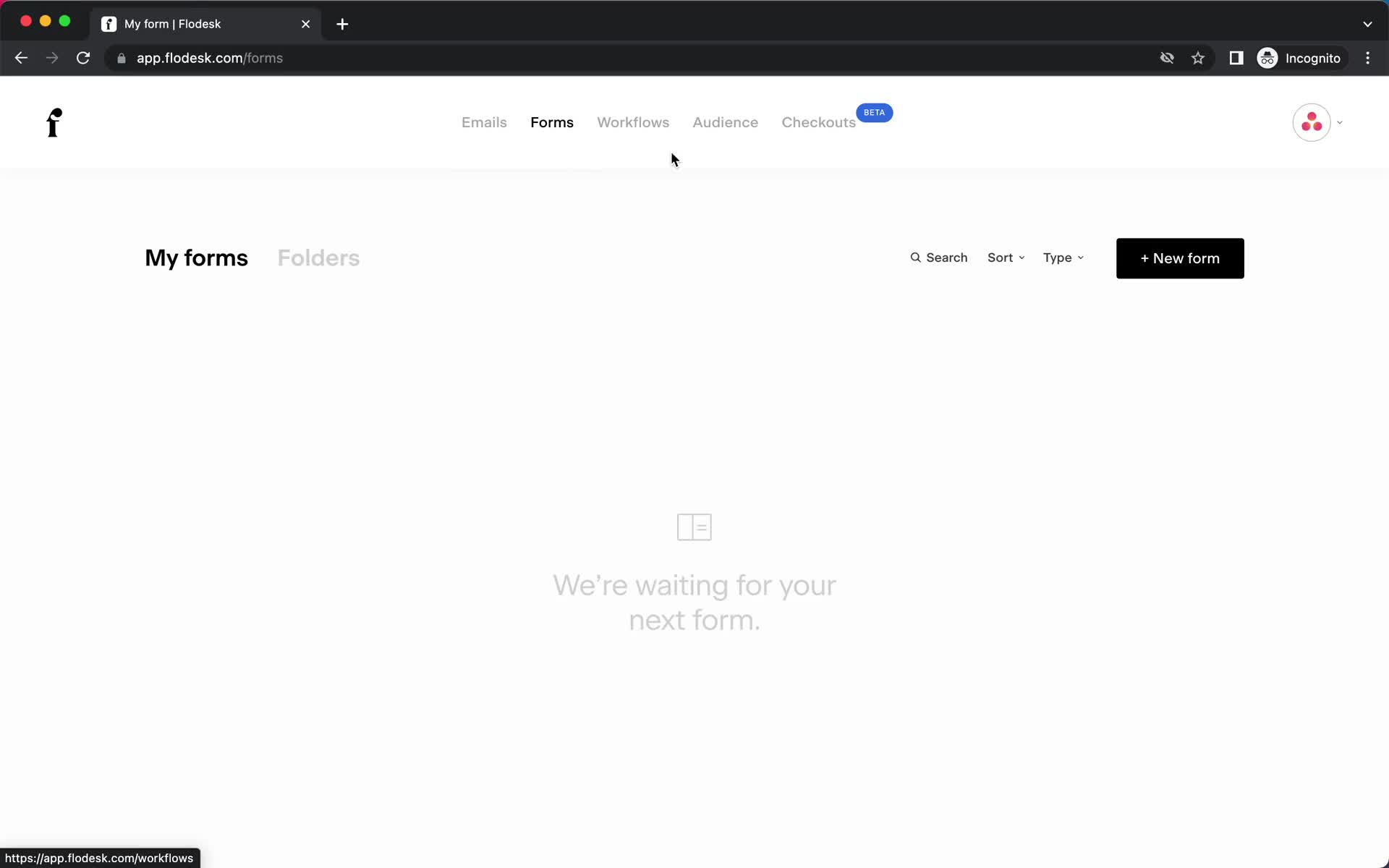The image depicts a screenshot of a Flowdesk user interface displayed within a web browser window. The browser itself features a sleek black background, adorned at the top left corner with three small, colored dots in red, yellow, and green. Adjacent to these dots, the text "My Forms" appears in a white font, followed by the word "Flowdesk," spelled out as F-L-O-D-E-S-K. Directly to the left of this text is the Flowdesk logo, resembling a stylized letter "F" within a white square.

The web address bar indicates the URL: app.flowdesk.com/forms, confirming that this is the forms section of the Flowdesk application. The main background color of the web page is a clean, bright white. At the top center of the page, a navigation menu is visible, containing the options "Emails," "Forms" (highlighted in bold to signify the current page), "Workflows," "Audience," and "Checkouts." "Checkouts" features a small rectangle with rounded corners and the word "Beta" inscribed in white, indicating that this feature is in its beta testing phase.

Below the navigation menu, on the left side of the screen, the header "My Forms" is presented in bold font, followed by the word "Folders" in a very light gray font. To the right side, there are options for "Search," "Sort," and "Type," with "Sort" and "Type" placed next to drop-down menu icons denoted by small, inverted gray triangles. Further to the right, a prominent rectangular button labeled "New Form" in white font, accompanied by a white plus sign, invites users to create a new form.

Centrally located on the page, a light gray message reads, "We're waiting for your next form," signaling an empty state and inviting the user to start creating forms.